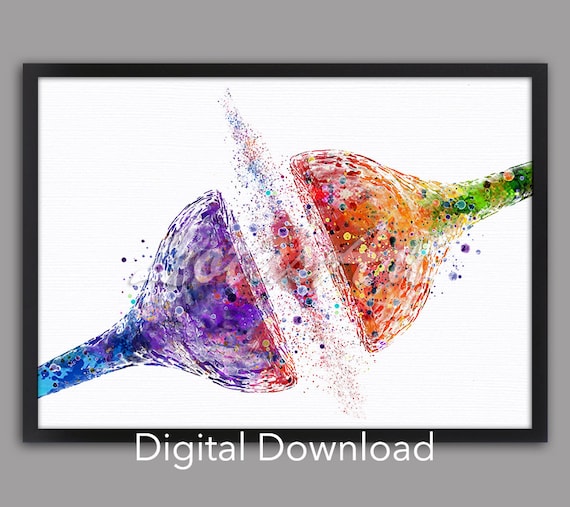The image is a vibrant digital painting set against a gray background, framed by a black border. It features an abstract portrayal resembling two splashes of water or wine glasses, creating an impression of a chemical reaction. The splashes are depicted in a spectrum of colors, starting with blue on the left and transitioning to purple, red, orange, and green towards the right. The colors meld explosively in the middle, with several particles dotting the area, adding to the dynamic effect. The lower half of the image contains white text reading "digital download."